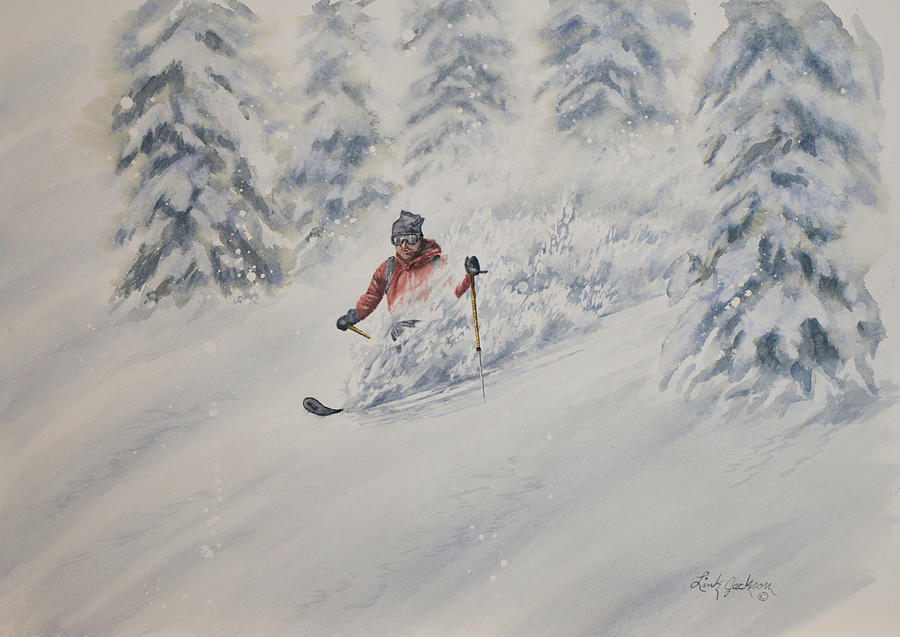This painting vividly captures a dynamic scene of a Caucasian male skier speeding downhill on a snow-covered slope. The skier, dressed in a striking red coat with the hood down, dons dark gray gloves, reflective goggles, and a black stocking cap. His motion is so swift that snow bursts up around him, nearly obscuring his legs and revealing only a partial view of one black ski. He grips ski poles, yellow at the top and transitioning to white near the base, with his left pole fully visible and the right one partially hidden by the flying snow.

Amidst the predominantly white canvas, flecks of color and detail emerge, including a visible gray strap across his shoulders. The serene winter backdrop features five to six snow-laden evergreen trees, their dark green needles partially visible through the heavy snow. Adding a personal touch, the artist "Linz Jackson" has signed the work in black at the bottom right. This composition beautifully blends the thrill of downhill skiing with the tranquil, snowy landscape, emphasizing the skier's confidence and speed.